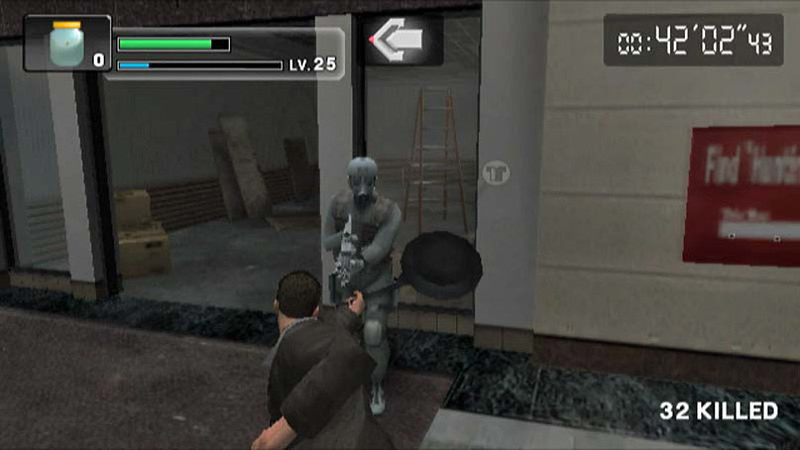In the foreground of a screenshot from a first-person shooter game, two characters are locked in dramatic confrontation. The background is dominantly composed of gray hues interspersed with touches of brown, giving the scene a stark, gritty atmosphere. On the upper left corner of the image, a blue jar with a yellow lid is prominently displayed; beside it, the number "0" is indicated. Below this, there are two status bars: a green one overlaying a thicker blue bar, with the text "LV.25" adjacent to them, denoting the player's level and health or shield status.

Continuing to the top right of the screen, a timer reads "00:42:02:43," possibly indicating how long the game has been running.

At the very center of the image stands a pivotal moment: a man, clad entirely in gray attire, aims his weapon directly at another man. The latter, dressed in a brown jacket and wielding a frying pan in his right hand, attempts to fend off his assailant with determined fervor. His brown hair frames a face focused on the immediate threat, adding human intensity to this virtual standoff.